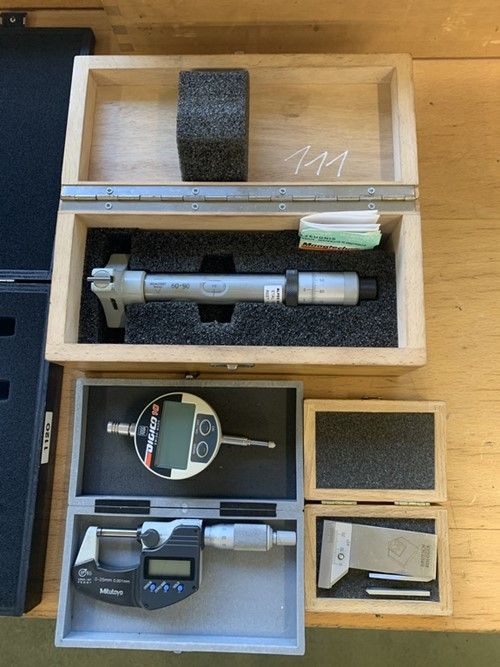The image shows three boxes of various sizes, all placed on a light wooden table that matches the color of the boxes. The largest box is positioned in the upper corner of the image and appears to be made from unfinished plywood. It is open to reveal both sides of the hinge. Inside, it has a foam insert and contains a large dull silver metal bar with ruler-type measurements and a twist area, suggestive of a measuring instrument. There's also a piece of folded paper next to a portable drill in the lower section. 

Beneath this large box are two smaller ones. The box on the bottom left is gray and contains a device resembling a durometer, which has a digital screen and metal posts extending from both the top and bottom. The smallest box, positioned next to the gray one, is a tiny wooden box identical in design to the large one. It houses a small silver tool, possibly another measuring instrument, resembling a caliper with a digital display. Velcro strips are visible in the lids of both wooden boxes, possibly for securing the tools. These boxes and tools appear to be intended for measurement and home construction uses.